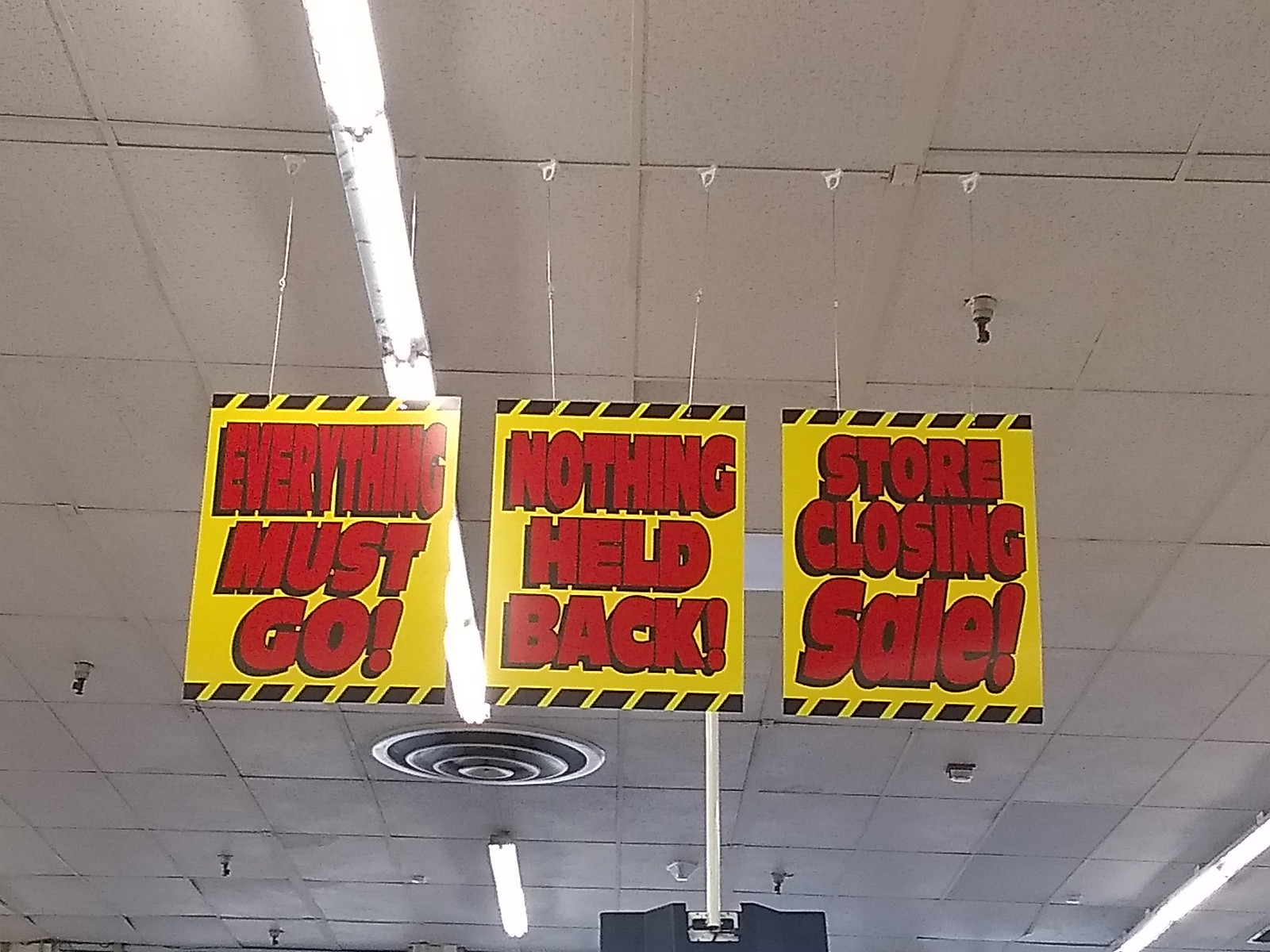The image depicts the ceiling of a store, characterized by white rectangular tiles arranged in a grid pattern formed by intersecting horizontal and vertical white lines typical of a drop ceiling. Slightly to the left center are rectangular-shaped industrial lights, flanked by several metal sprinklers poised to activate in the event of a fire.

Prominently hanging from the ceiling are three rectangular signs, each suspended by two silver wires attached to the top corners. These signs share a consistent design theme with yellow backgrounds and prominent black stripes along the top and bottom edges. Each sign features bold red lettering. The leftmost sign reads, “EVERYTHING MUST GO!” The middle sign states, “NOTHING HELD BACK!” The rightmost sign declares, “STORE CLOSING SALE,” with "SALE" uniquely formatted with a capital "S" followed by lowercase "a-l-e." All text is in capital letters, except for “SALE,” and each phrase is punctuated with an exclamation point, emphasizing the urgency of the sale.